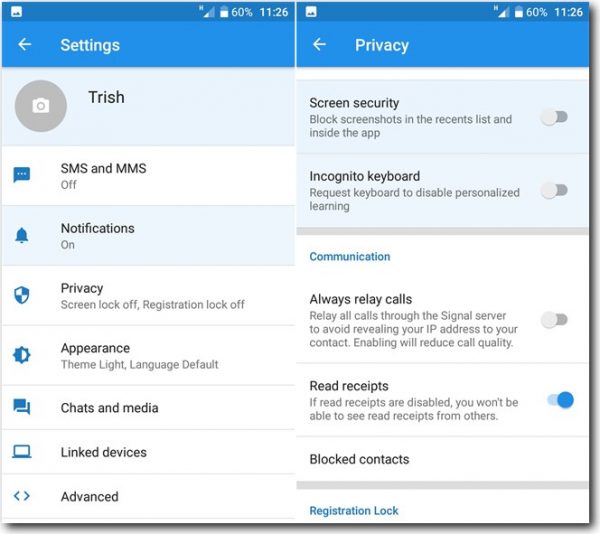"Two screenshots are presented side-by-side, both captured at 11:26 with a battery percentage of 60%. The screenshots feature two distinct sections: 'Settings' on the left and 'Privacy' on the right, each identified by a bright blue header with a back arrow.

**Left Screenshot: Settings**
- Below the header, there's a placeholder for a profile photo, currently displaying a camera icon.
- The user, Trish, has the following settings displayed in a list:
   - SMS and MMS: Off
   - Notifications: On
   - Privacy
   - Screen Lock: Off
   - Registration Lock: Off
   - Appearance: Light Theme
   - Default Language
   - Chats and Media
   - Link Devices
   - Advanced

**Right Screenshot: Privacy**
- Screen Security:
   - Block Screenshots in Recent List and Inside App: Off
- Incognito Keyboard:
   - Request Keyboard to Disable Personalized Learning: Off
- In blue text, Communication Settings:
   - Always Relay Calls: Off (Relays all calls through server to hide IP address; may reduce call quality)
- Read Receipts: On (Disabling prevents you from seeing others' read receipts)
- Blocked Contacts
- Registration Lock in blue text below

The overarching theme of both screenshots includes bright blue accents for headers, icons, and specific text elements, providing a cohesive visual design emphasizing certain areas within the settings and privacy options."